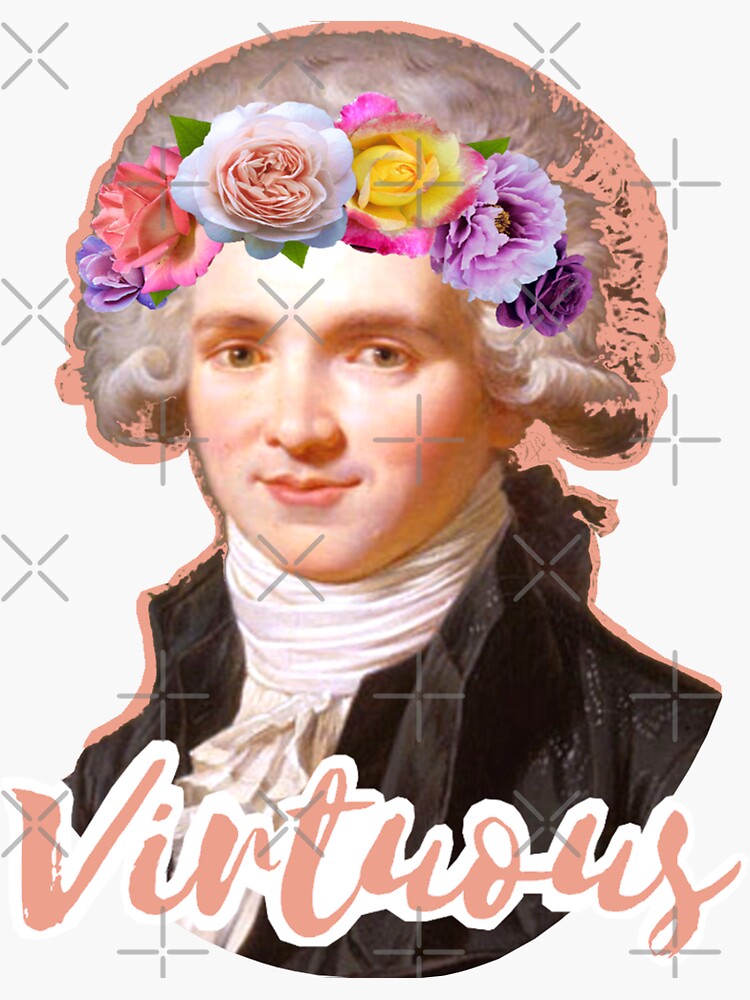The image depicts a pixelated and stylized illustration of a late 18th-century bust, centrally positioned, either resembling a young man or woman adorned in period attire. The figure wears a distinctive black or dark jacket paired with a white, frilly scarf around the neck. The powdered wig or grey, fluffy hair is lavishly adorned with a variety of colorful flowers including white, yellow, purple, and pink blooms, totalling about six different flowers. These adornments create an ornate, almost headdress-like appearance. The artwork is accentuated with a salmon-colored border. The word "Virtuous" is prominently displayed in large, stylized pink letters with a white border across the chest of the bust. The background is primarily white, though multiple layers, possibly transparent watermarks shaped like crosses and plus signs, add complexity to the visual field. Despite a high level of detail in the depiction, the overall image is noted to be somewhat blurry and pixelated, potentially suggesting a digital rendering or reproduction.